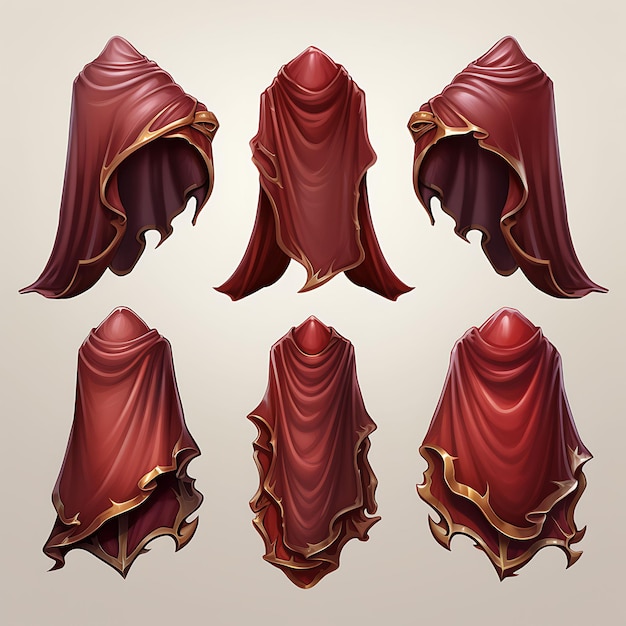The image is a detailed, colored digital illustration that is essentially square and set against a light gray background, without a distinctive border. It features six red cloaks or robes adorned with gold trim, arranged in two rows of three. The top row depicts designs resembling helmets or headpieces viewed from multiple angles, showcasing the ornate and domed top with a pointed tip. The bottom row presents the cloaks in full, with the central piece being the thinnest and flanked by two slightly wider versions. The artist's rendition highlights the texture and drape of the fabric, emphasizing the soft and nimble qualities through visible curvature lines. The illustrations appear as concept designs, potentially for a video game or role-playing game, providing a comprehensive view of both the front, back, and sides of the cloaks.